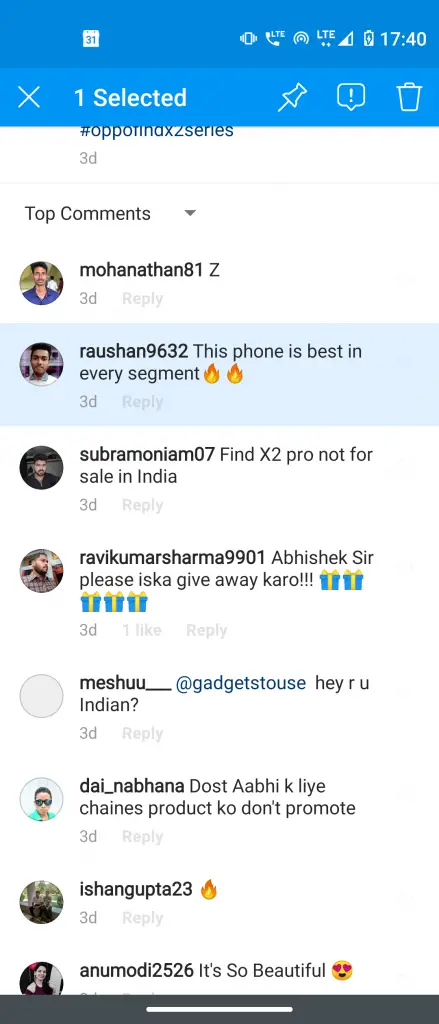In the image, the topmost section features a dark blue rectangular header aligned towards the left. Within this header, there is a small white calendar icon displaying the number "31" in blue text. Positioned immediately to the right, the icon representing a phone on vibrate is visible. Next to this, a stylized phone icon appears with the top piece tilted left and the bottom piece tilted right, accompanied by the text "LTC" or "LTE" at the top. Right beside this, several curved signal lines are visible, indicating signal strength.

Further right, the letters "LTE" are prominently displayed in capital letters with two downward-pointing arrows situated nearby. Proceeding to the right, there are four out of five signal bars, suggesting strong network coverage. Next to these bars, a battery icon with a charging symbol is present, and to its right, the time is displayed as "17:40" in white text.

Below this, there's a slightly thinner header in a lighter blue shade. On the far left of this header, a thin white "X" is displayed. Immediately to its right, the bold text "One selected" is visible. Following this, there's a push pin icon angled towards the bottom left. Next to this push pin, there's a message bubble containing an exclamation point, and further to the right, a small trash can icon is seen.

Beneath this, partially cut off, there seems to be a hashtag that appears to read "OPPOFINAX2 series." Underneath this hashtag, the text "3D" (likely indicating "three days ago") is printed in small gray letters on the left. Below this text, a very faint light gray divider line is visible. On the left side of this divider, there is a black drop-down menu displaying "Top comments," and to the right of this menu, a gray arrowhead is pointing downwards.